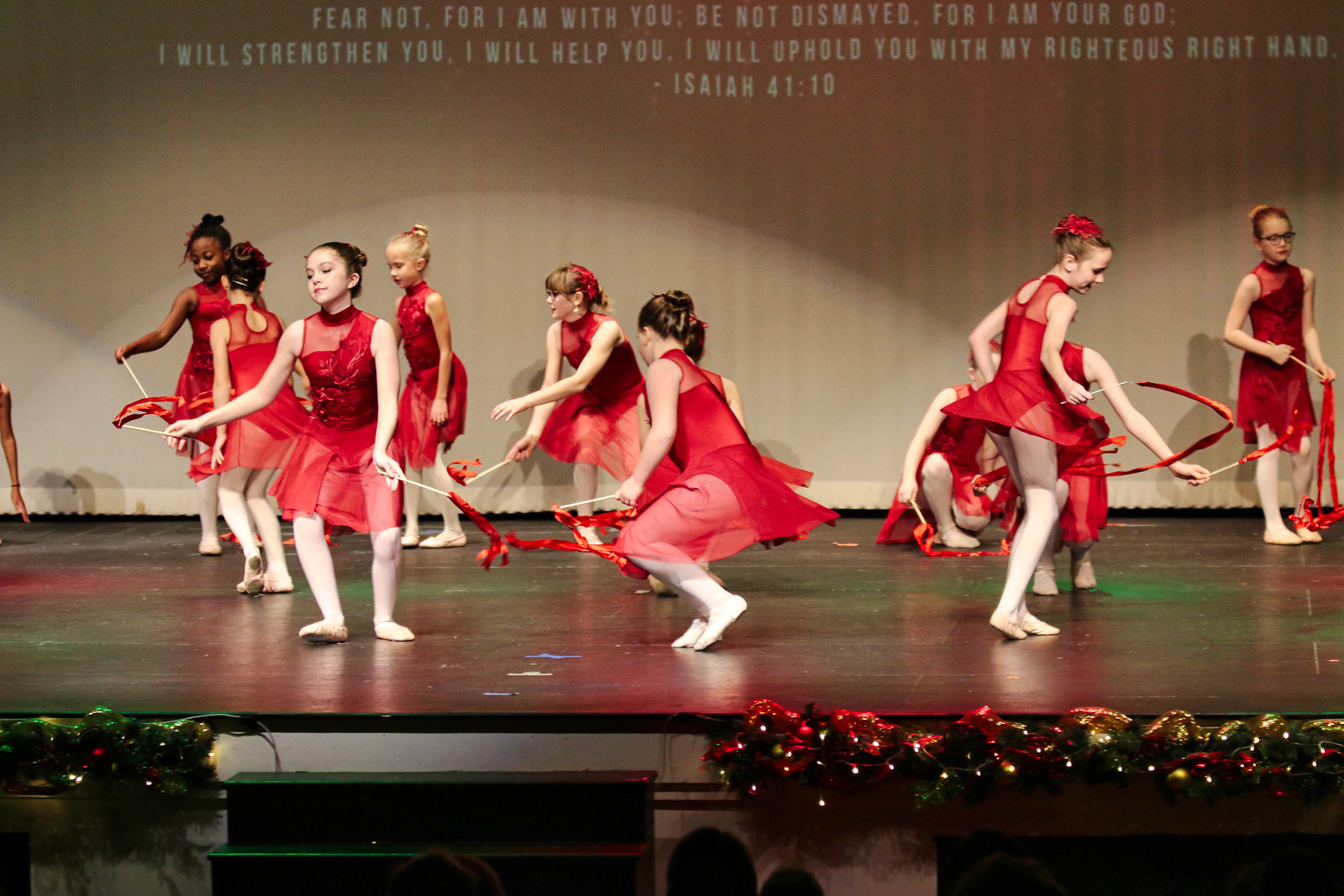The image depicts a group of ten young female dancers, part of a children's dance corps, performing a choreographed routine on stage. Each girl is dressed in a red ballet outfit and white ballet shoes, with their hair neatly styled in buns; one of the girls is notably wearing glasses. They hold white wands tipped with red, and are arranged in varying poses as they gracefully execute a circular dance pattern. The stage features Christmas decorations at the front, hinting at the festive nature of the performance, while the wooden stage floor contrasts with the light beige curtain backdrop. Above the dancers, a message is prominently displayed on the curtain: "Fear not, for I am with you. Be not dismayed, for I am your God. I will strengthen you, I will help you, I will uphold you with my righteous right hand. Isaiah 41:10." The scene is well-lit, enhancing the visibility of the dancers' expressions and movements. In the foreground, elements of the audience and additional stage decorations are visible, adding to the lively and joyous atmosphere of the event.